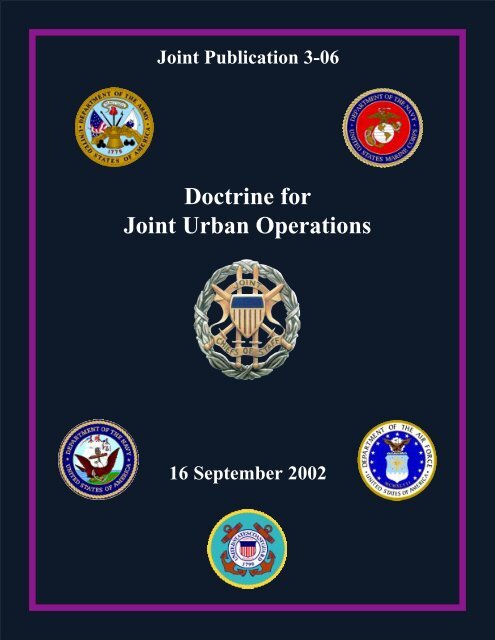The cover of the manual titled "Joint Publication 3-06: Doctrine for Joint Urban Operations," dated 16 September 2002, features a dark navy blue background with a purple, magenta-bordered frame. Central to the cover is an emblem with a shield depicting the U.S. flag, encircled by a silver, rope-like wreath, and accompanied by the text "Joint Chiefs of Staff." At the top of the cover, the title is displayed in white font. In the upper left corner is the emblem of the Department of the Army, featuring an eagle with the American flag and another white flag behind its wings, encircled by the text "United States of America, Department of the Army." On the upper right side, there's the emblem of the United States Marine Corps, Department of the Navy, displaying a globe with golden continents on a red background. At the bottom, there are three additional seals: the Department of the Navy with a boat, the Department of the Air Force with a blue background and an eagle, and an unclear seal in the middle.